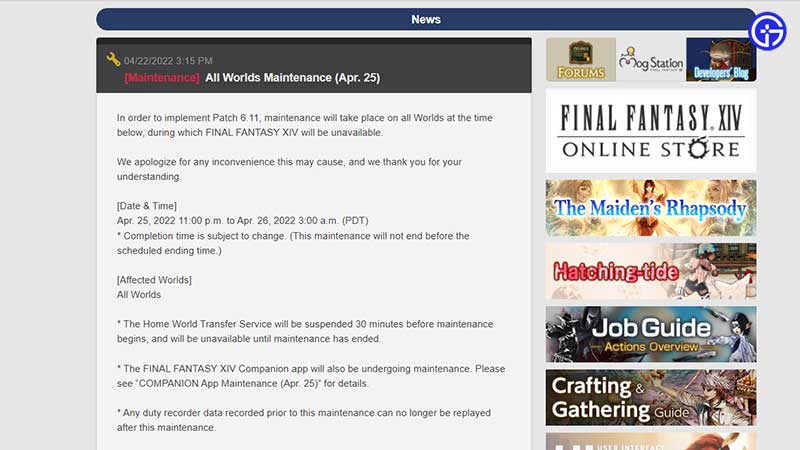The web page is divided into two columns. At the top of the page, there is a prominent, rounded button displaying the word "News" in white text. The left column is dedicated to informing users about an upcoming server maintenance for Final Fantasy XIV, scheduled for April 25th. The alert is presented on a gray background with black text and reads: "In order to implement patch 6.11, maintenance will take place on all worlds at the time below during which Final Fantasy XIV will be unavailable." 

The right column features a series of buttons that provide quick access to various resources. These include "Forums," "Mogstation," "Developer Blog," and a button with a white background and black text featuring the Final Fantasy XIV Online Store logo. Below these buttons, there's a visually appealing section titled "The Maiden's Rhapsody," designed predominantly in yellow and brown, with a gradient blue text. Further down, there's a section titled "Hatching Tide" in red, followed by additional game-related links such as "Job Guide: Actions Overview" and "Crafting and Gathering."

The overall design highlights critical information while offering easy navigation to other areas of interest within the game’s community and resources.